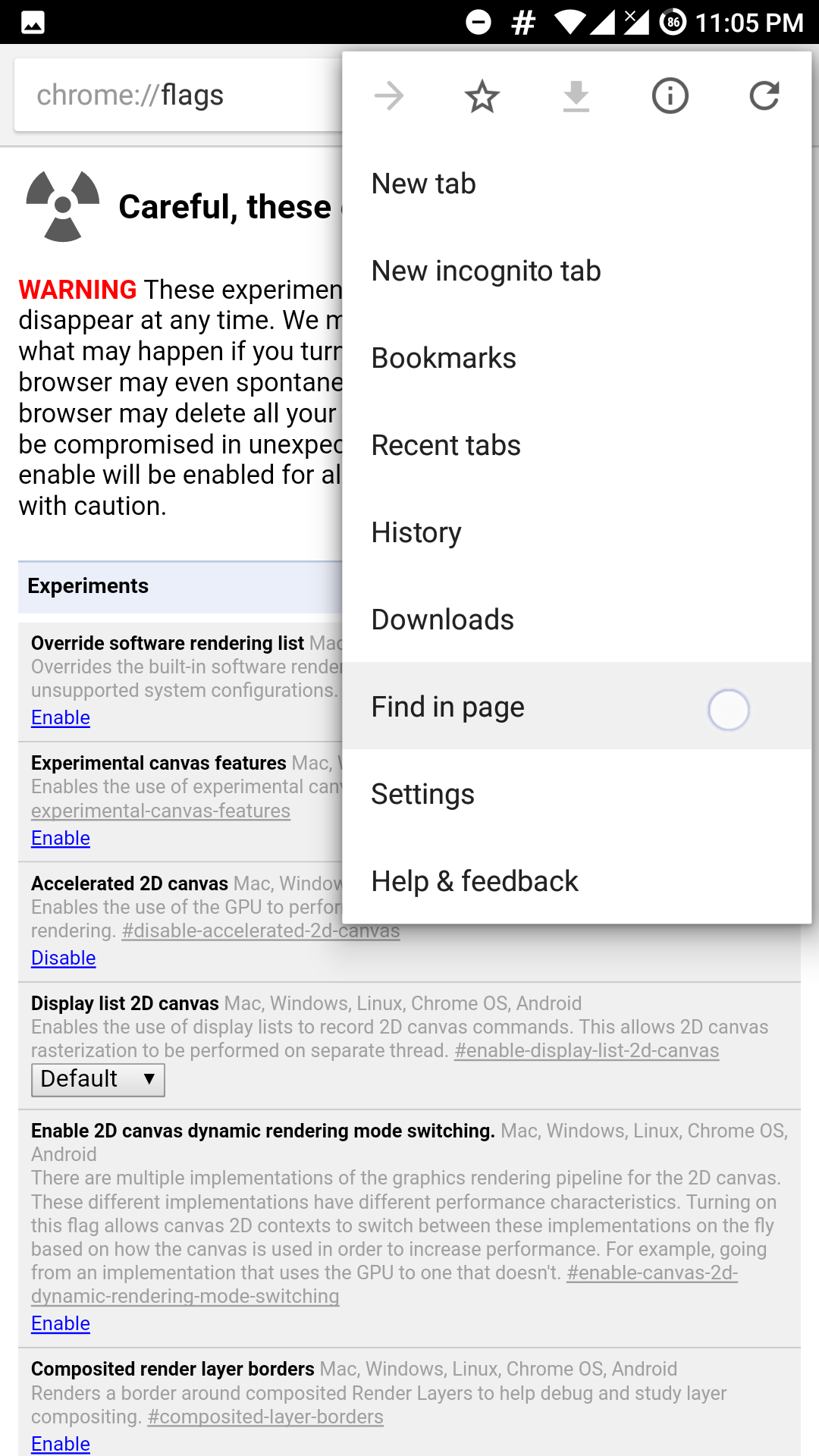The image is a screenshot of a part of a website viewed on a mobile phone. The upper left corner features a gallery icon, while the entire top right side shows various cellphone icons, including a Wi-Fi icon, a signal indicator, and a clock displaying the time as 11:05 PM. Below this, the browser tab menu is open, displaying several icons including a star, a download arrow, another unidentified icon, and a refresh icon toward the right.

The open tab menu lists several options:
- New tab
- New incognito tab
- Bookmarks
- Recent tabs
- History
- Downloads
- Find in page (highlighted in gray)
- Settings
- Help and feedback

On the left side at the top of the screen is the URL bar. Below it, partially visible text reads "careful, these" followed by obscured content. Next to this text is a red warning icon and a paragraph of black text.

The lower section of the screenshot displays various settings that can be enabled or disabled. Each setting is labeled in black and accompanied by a brief description. The words "enable" and "disable" are in blue text. There is also an option labeled "default."